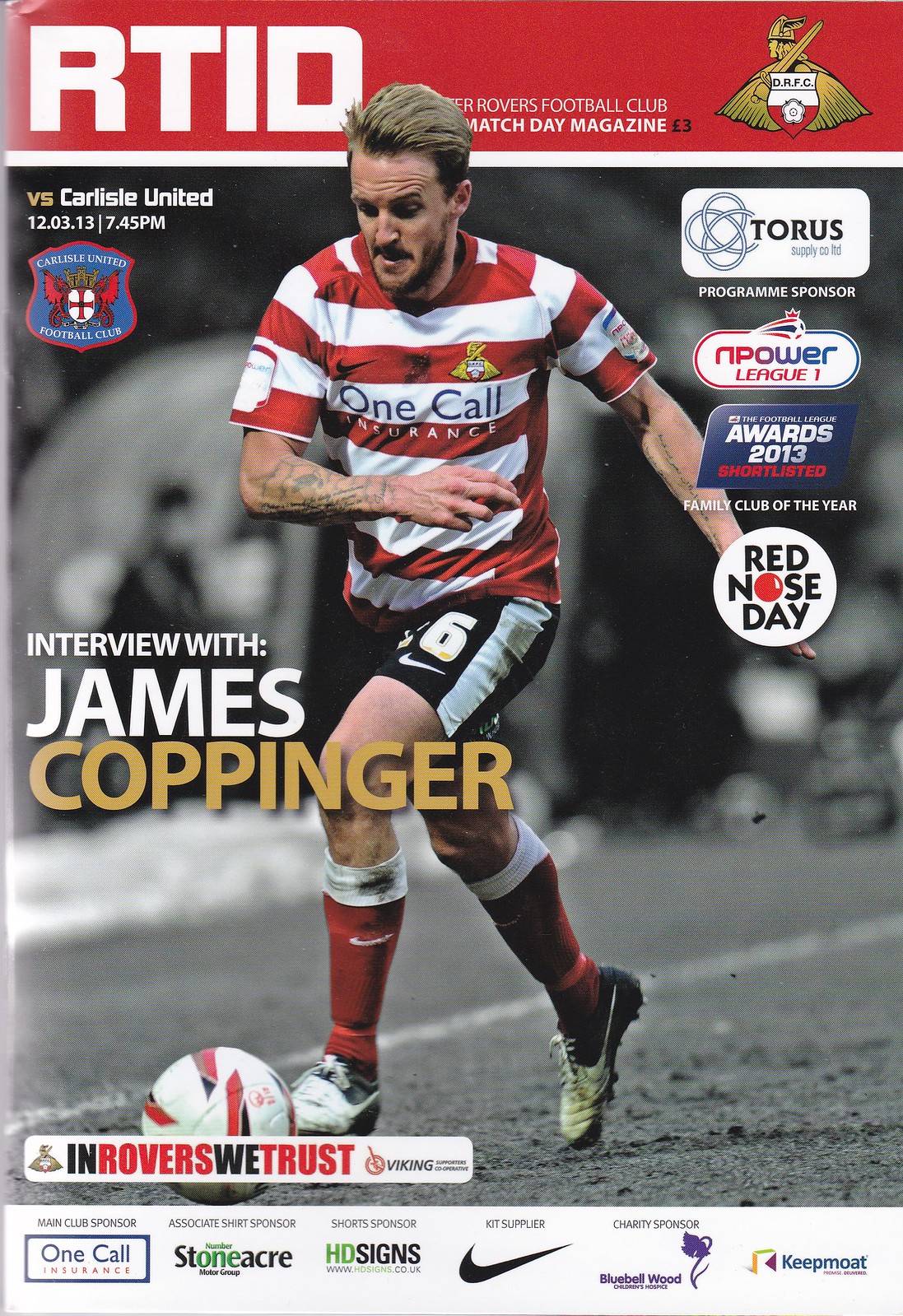The cover of the Match Day Magazine for the soccer game on December 3rd, 2013, features a dynamic action shot of a player mid-match, distinguished by his red and white striped jersey, black shorts with a white stripe, and red socks. This player is likely James Coppinger, who is highlighted for an interview within the magazine. He has tattoos on both forearms, sports a short blond beard, and is running to the left, kicking a soccer ball with his left foot. The black and white background contrasts with the vivid colors of his uniform. 

The title reads "RTID" at the top, with "Something Rovers Football Club" next to it on the banner, indicating the publication is a match day magazine for the 'Rovers versus Carlisle United' game, priced at three pounds. The match is set to commence at 7:45 p.m. Featured logos are present, likely representing sponsors such as Torres Supply Co Ltd, Bluebell Wood Children's Hospice, and main club sponsor 'One Call Insurance', displayed prominently on the white part of the player's jersey. Other sponsors mentioned include Stoneacre Motor Group, HD Signs, Nike, and Power League One, Family Club of the Year, among others, underscoring strong community and commercial support behind the event.